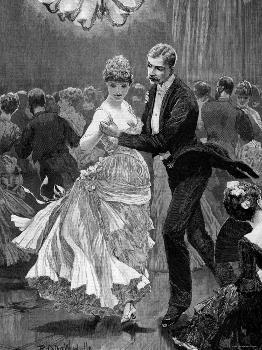In this detailed black-and-white drawing, a lavish ballroom scene unfolds, showcasing multiple elegantly dressed couples engaged in dance. The foreground features a prominent couple: a woman in a sleeveless, thin-strapped dress with a low neckline, her flowing skirts cascading to her ankles as she gracefully holds the hands of her partner. Her hair is styled in an intricate curly bun. Her partner, a distinguished man with a mustache, is clad in a black tuxedo jacket, white button-up dress shirt, black pants, and black shoes, gazing down as they twirl. Above them, a partially visible chandelier hangs from the ceiling, casting light onto the lightly shaded gray wall in the background, which is adorned with a curtain on the upper right side. Surrounding the main couple, similarly dressed men and women fill the background, creating a lively atmosphere of a grand black-tie event. The men predominantly wear dark suits, while the women don elegant gowns, their vintage attire evoking a bygone era. The scene is completed with faint text at the bottom and a gray-tinted floor, capturing the timeless elegance and social grace of the ballroom setting.